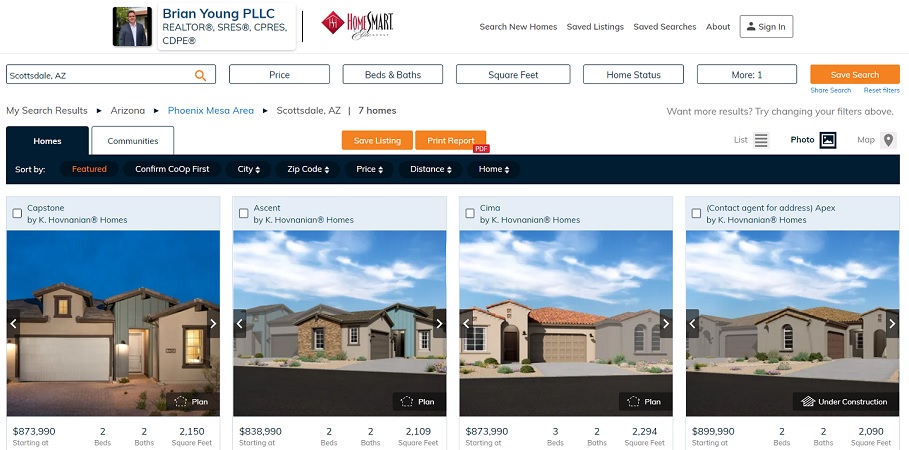Caption:

"Screenshot from the Brian Young, PLLC Realtors real estate website featuring a professional portrait of Brian Young in a suit jacket and white shirt. The website header includes the 'HomeSmart' logo with a red diamond emblem, and offers options to 'Search New Homes,' 'Save Listings,' 'Save Searches,' and 'About.' A white sign-in box with a black profile image is prominently displayed. Under the search bar, various filters like price, number of beds and baths, square footage, home status, and more can be adjusted, with 'Scottsdale, Arizona' shown as the example search location. Users can save or share searches and a reset button is available. Below, the 'My Search Results' section lists search outcomes with options to focus on different regions like 'Phoenix' and 'Mesa.' Results for 'Scottsdale, Arizona' show seven listings, with categories for 'Homes' in black and 'Communities' in white. Each home listing includes details like price, square footage, and number of beds and baths. The layout features modern and ranch-style homes with accompanying images and options to save the listing or print a report."